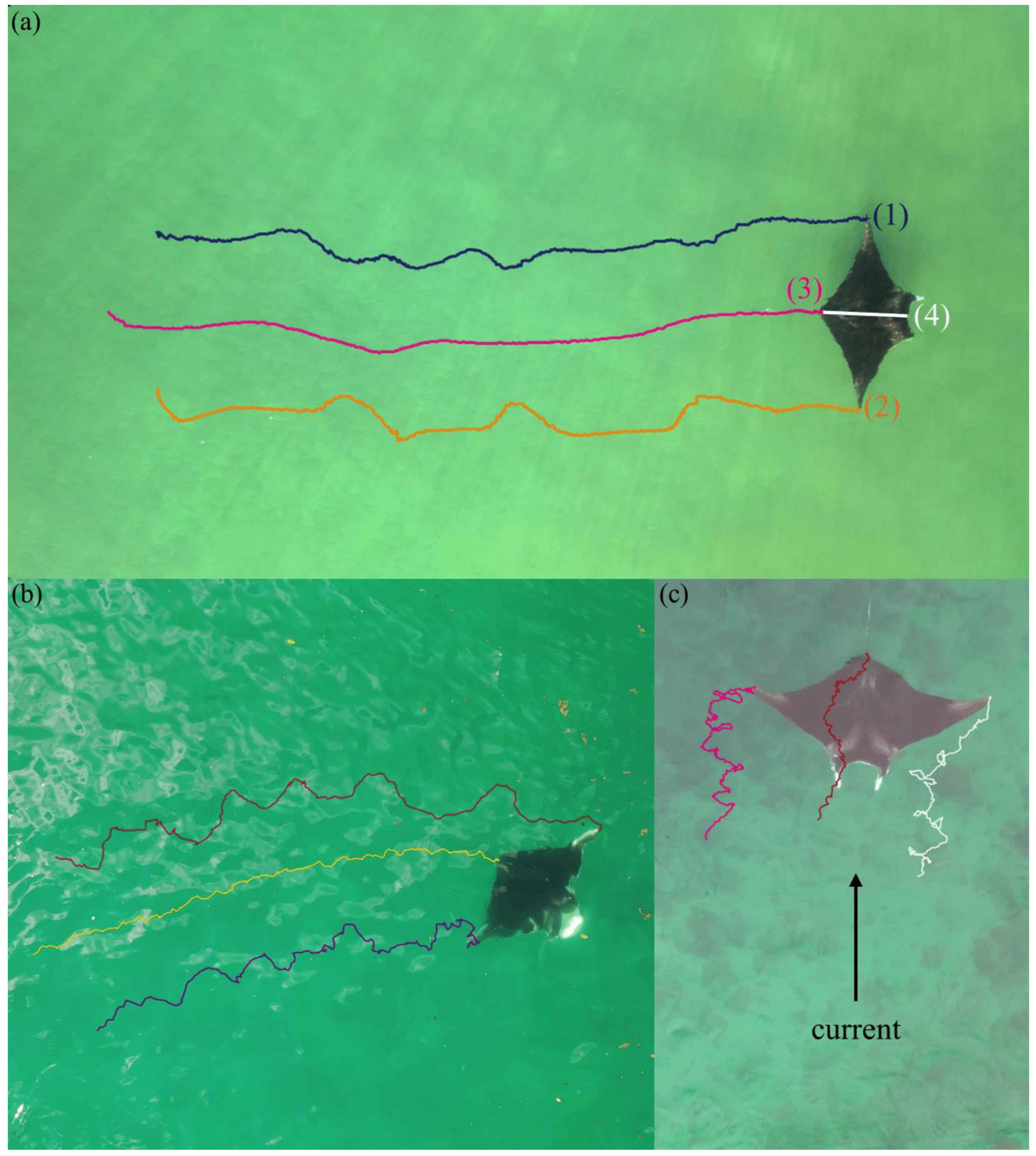The graphic features three images labeled A, B, and C, each displaying a top-view photograph of a black stingray swimming in water. The photographs are arranged with one at the top (A), one at the bottom left (B), and one at the bottom right (C).

In Image A, the stingray is swimming to the right in light green water. Its body is on the right side of the image, and it has three colored lines emanating to the left: blue (1), pink (3), and yellow (2). Additionally, there are numbers (1, 2, 3, 4) in various colors next to its body, and the letter "A" is marked in black at the top left corner.

In Image B, the stingray appears in dark green water, with three colored lines – red, yellow, and blue – surrounding it. The letter "B" is placed in the top left corner, with no additional numbers present around the stingray.

In Image C, the stingray is featured in bluish water. Three lines, pink, red, and white, radiate around it. There's also a black arrow beneath the stingray labeled "current." The letter "C" is written in the top left corner of this image. 

Overall, the graphic highlights the stingray's movement and possibly monitors the water currents through varied graphical annotations in each image.